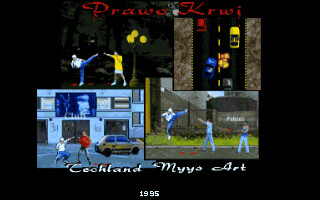This multi-paneled image resembles various video game screens, each vividly portraying scenes of action and combat.

**Top Left Panel**: Two figures are locked in combat, assuming dynamic fighting stances. One character, dressed in a white hat, white shirt, blue pants, and white shoes, has their leg extended in a high kick aimed at their opponent's head; however, the kick misses by several feet. The opposing character, clad in a yellow t-shirt, white shorts, and white shoes, counters with a punch directed toward the kicking foot, also missing by about a foot. Behind them are three round, glowing lights illuminating the intense scene.

**Top Right Panel**: This section displays a busy road scene. The black asphalt road, distinguished by a yellow dashed line down its center and brown embankments on either side, is teeming with four cars in motion. A blue car leads the convoy, followed by a yellow car, a red car, and a black car, all heading in the same direction.

**Bottom Left Panel**: Another combat scenario is depicted here. The character in the white hat, white shirt, and blue pants is now crouching and launching a punch toward an adversary sporting a red top and light-colored pants, but the punch falls short by a couple of feet, creating a palpable tension as the two figures engage.

**Bottom Right Panel**: The final scene captures the white-hat character mid-air, executing a powerful jump kick a few feet off the ground. Their kick soars over the head and several feet away from a new opponent wearing a light blue shirt and pants, who appears to be throwing a punch upward toward the airborne fighter. A third character, dressed in a blue tank top and light blue pants, stands in the background, possibly discharging a weapon, as evidenced by a red flare emanating from their position. There is also an unsettling presence of blood on the ground, adding to the dramatic intensity of the scene.

Overall, the image masterfully conveys a sense of vigorous action and suspense, capturing the viewer’s attention with its vivid and dynamic compositions.